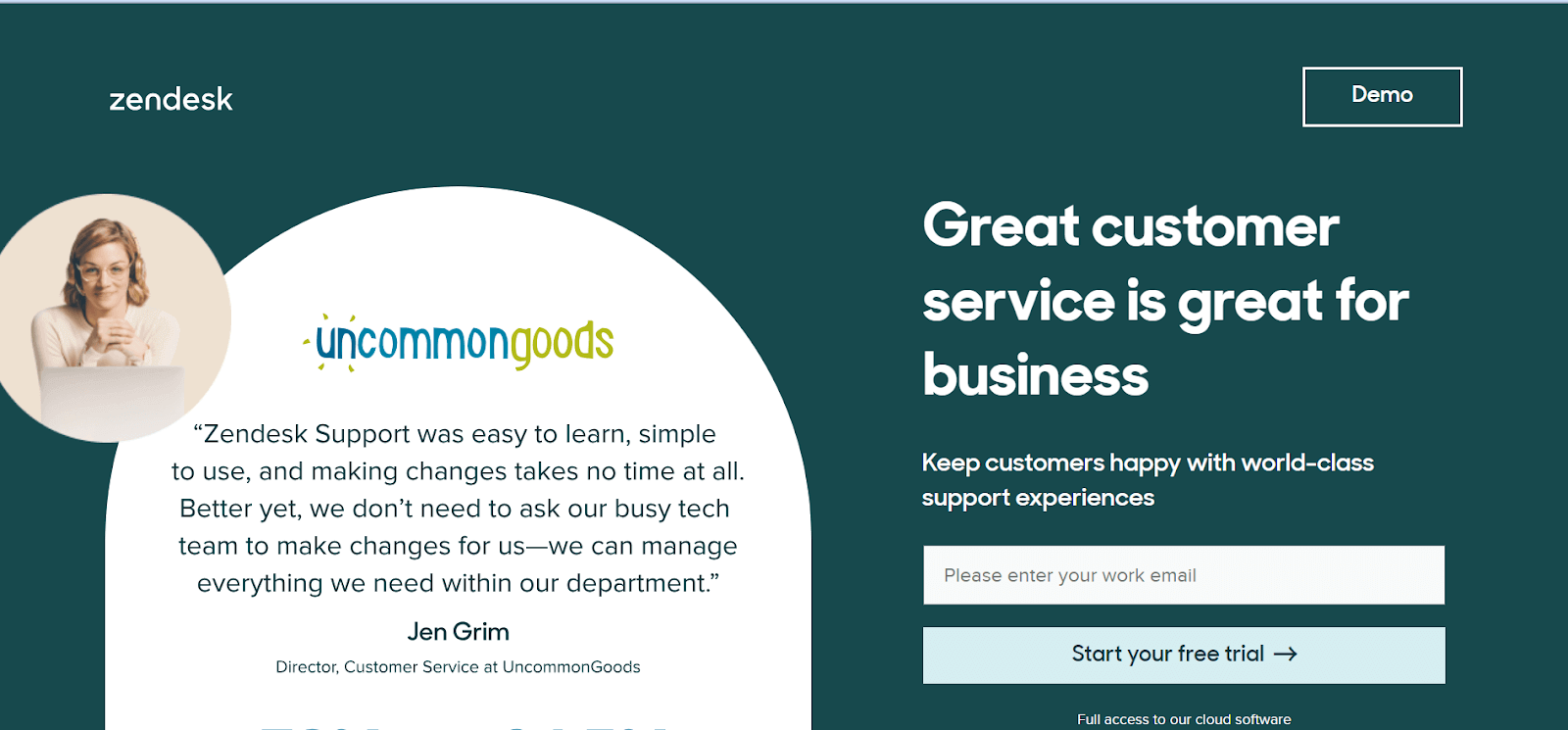The webpage you're viewing appears to offer a customer service solution aimed at enhancing client satisfaction. The background is a dark green color, accented with white elements and bubbles containing images. 

In the top left corner, the company name "Zendesk" is prominently displayed in white text. Just below, there's a beige bubble featuring a young Caucasian woman with blondish-red hair and glasses. She is wearing a beige shirt and appears to be standing at a white podium.

To the right of this image, there is a white, gravestone-shaped icon that encloses a blue and green logo reading "Uncommon Goods" (with "Uncommon" in blue and "Goods" in green). Beneath the logo is a testimonial in black text, stating: "Zendesk support was easy to learn, simple to use, and making changes takes no time at all. Better yet, we don't need to ask our busy tech team to make changes for us. We can manage everything we need within our department. Jen Grimm, Director and Customer Service at Uncommon Goods."

Further to the right, there's a headline that reads, "Great Customer Service is Great for Business - Keep Customers Happy with World-Class Support Experiences."

Below this headline, a white text box prompts users to "Please enter your work email," accompanied by a blue button that says "Start your free trial." An additional line underneath reads, "Full access to our cloud software."

In the top right corner, there is a rectangular button labeled "Demo."